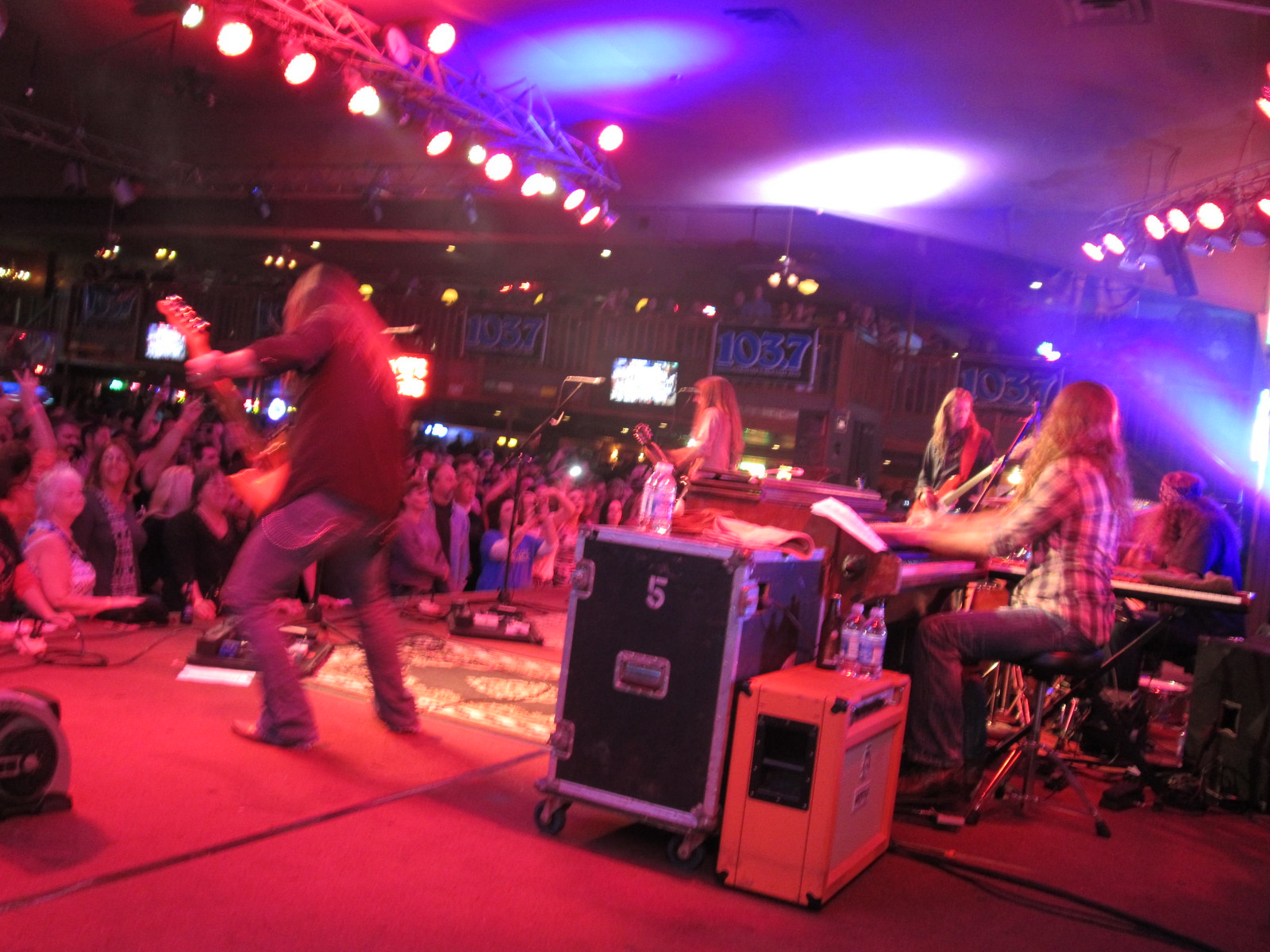This captivating photograph captures the energy and atmosphere of a live performance inside a bustling bar venue, taken from a vantage point behind and slightly to the left of the stage. The center of attention is the band, composed of four long-haired musicians, each engrossed in their musical roles. 

On the left side of the stage stands a guitarist in a long-sleeve t-shirt and jeans, strumming his instrument with fervor. To the right, a bassist in a dark brown shirt and blue pants plays steadily. At the center back of the stage, a keyboardist sits behind their instrument, singing into a microphone. They have long red hair and are dressed in a plaid shirt and jeans. Another guitarist, positioned further to the right, wears a white shirt and joins in the harmony.

The stage is awash with vibrant red, pink, and blue lighting from a rig centered above, casting a dynamic glow over the performers and enhancing the mood of the venue. In the background, "1037" is illuminated in blue, adding a unique touch to the setting. In front of the stage, a diverse crowd jams out, with many individuals raising their hands and cheering in unison to the music. The mix of the detailed lighting, the lively audience, and the passionately engaged band collectively bring this image to life.